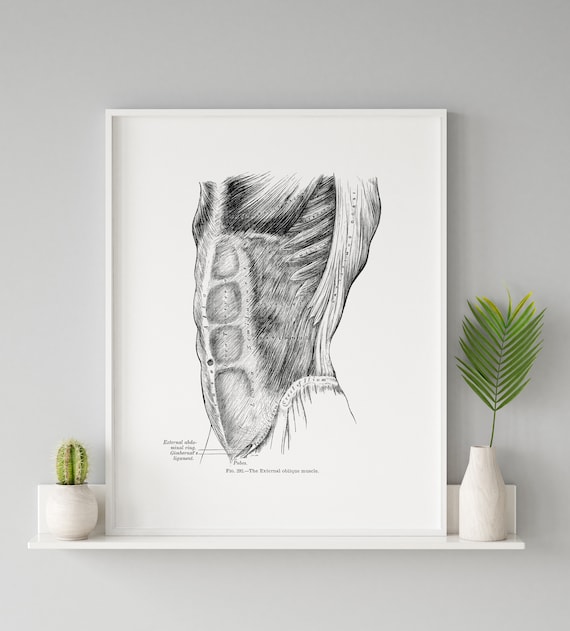This black-and-white hand-drawn ink sketch, framed in white, is an intricate depiction of human abdominal anatomy. The drawing, which resembles an old medical diagram, meticulously illustrates the abdominal muscles, complete with dashed lines and arrows highlighting various muscle groups and anatomical features. The artwork, primarily in black ink with some gray shading, reveals the muscular structure under the skin, focusing on the prominent 'six-pack' abs.

The framed illustration rests on a narrow white shelf against a gray wall. On the left side of the shelf, a small, spiky cactus sits in a white pot, adding a touch of greenery. On the right end, a white vase contains a single palm frond, offering a striking contrast to the meticulous detail of the anatomical sketch. The shelf is just wide enough to accommodate the framed drawing and the two plant containers, creating a balanced and aesthetically pleasing display.